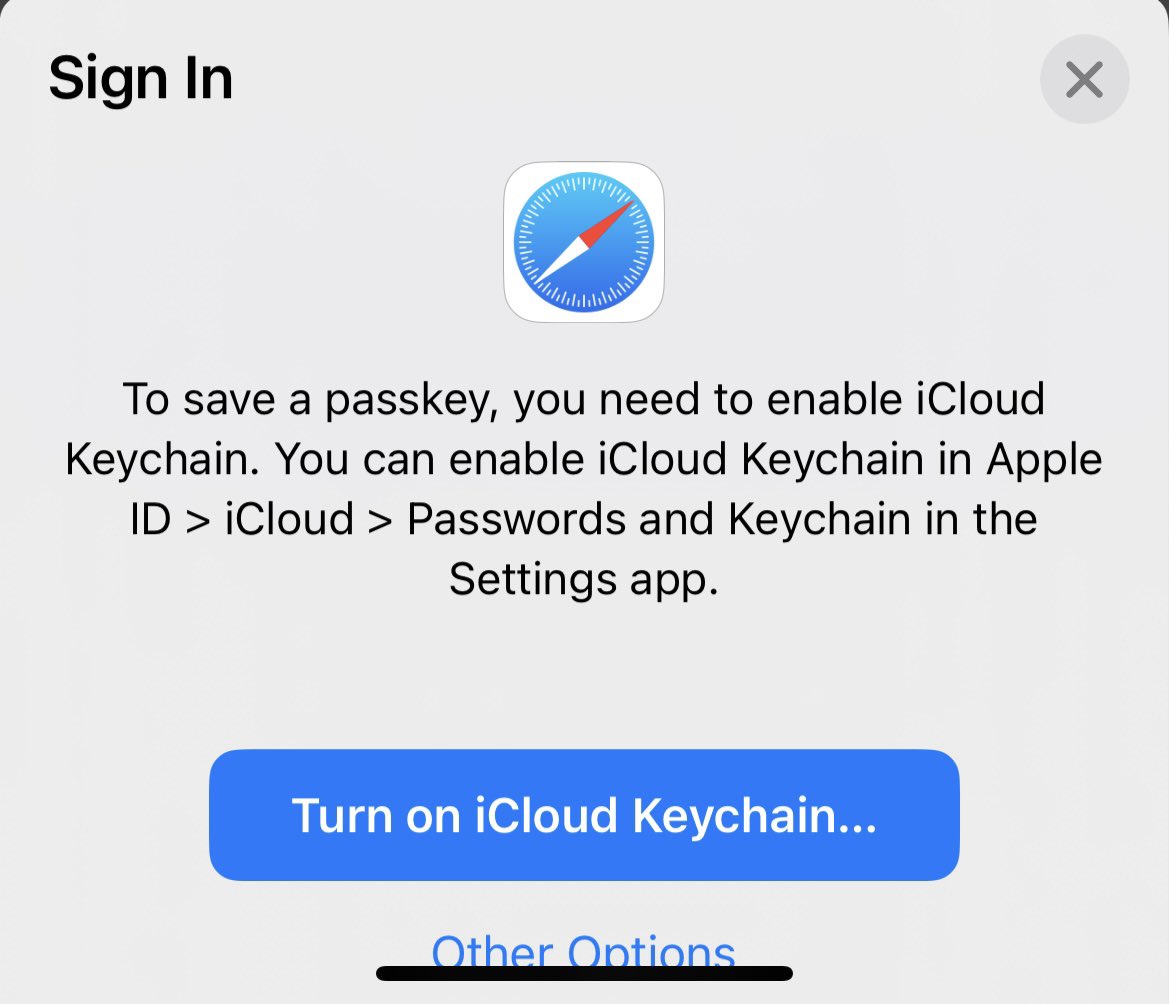This image features the sign-in page of the Apple Safari app. Dominating the center of the page is the iconic Apple Safari app logo. Below the logo, the page displays a message: "To save a passkey, you need to enable iCloud Keychain. You can enable iCloud Keychain in the Settings app under Apple ID > iCloud > Password & Keychain." Additional instructions are present beneath this message, appearing as: "Turn on iCloud Keychain," with the phrase "other options" prominently underlined in black. The page is set against a clean, minimalistic background, typical of Apple's design aesthetic.